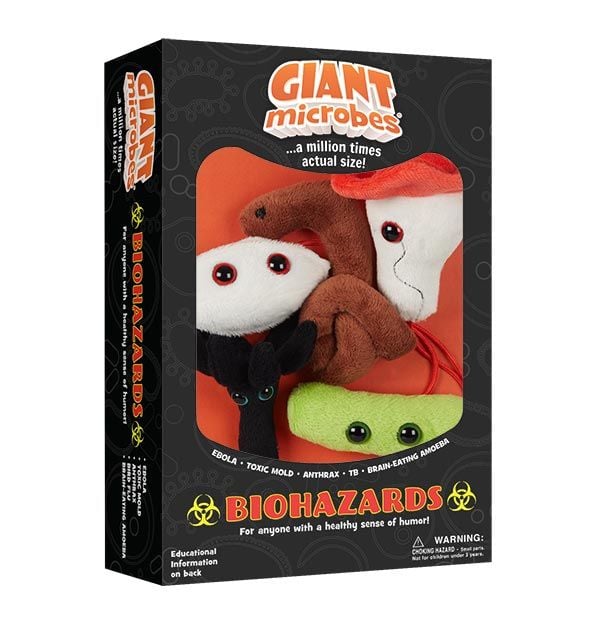The photograph showcases a product box set of educational plush toys named "Giant Microbes," displayed against a seamless white background, giving an edited appearance. The black, rectangular box, longer on its left and right sides, features a clear window through which several colorful plushies can be seen. Above the window, an orange text on a white background reads "Giant Microbes," followed by white text stating "a million times actual size." Below the window, there is a list of the included microbes: Ebola, Toxic Mold, Anthrax, TB, Brain Eating, and MOBA, with a reference to Staphylococcus aureus in one of the captions. The box and its contents are primarily black with various red, white, yellow, and green accents on the plushies. Despite the humorous and unusual nature of the product, it serves an educational purpose, likely designed to teach children and others about different microbes and infectious diseases through visually engaging, exaggerated plush representations.